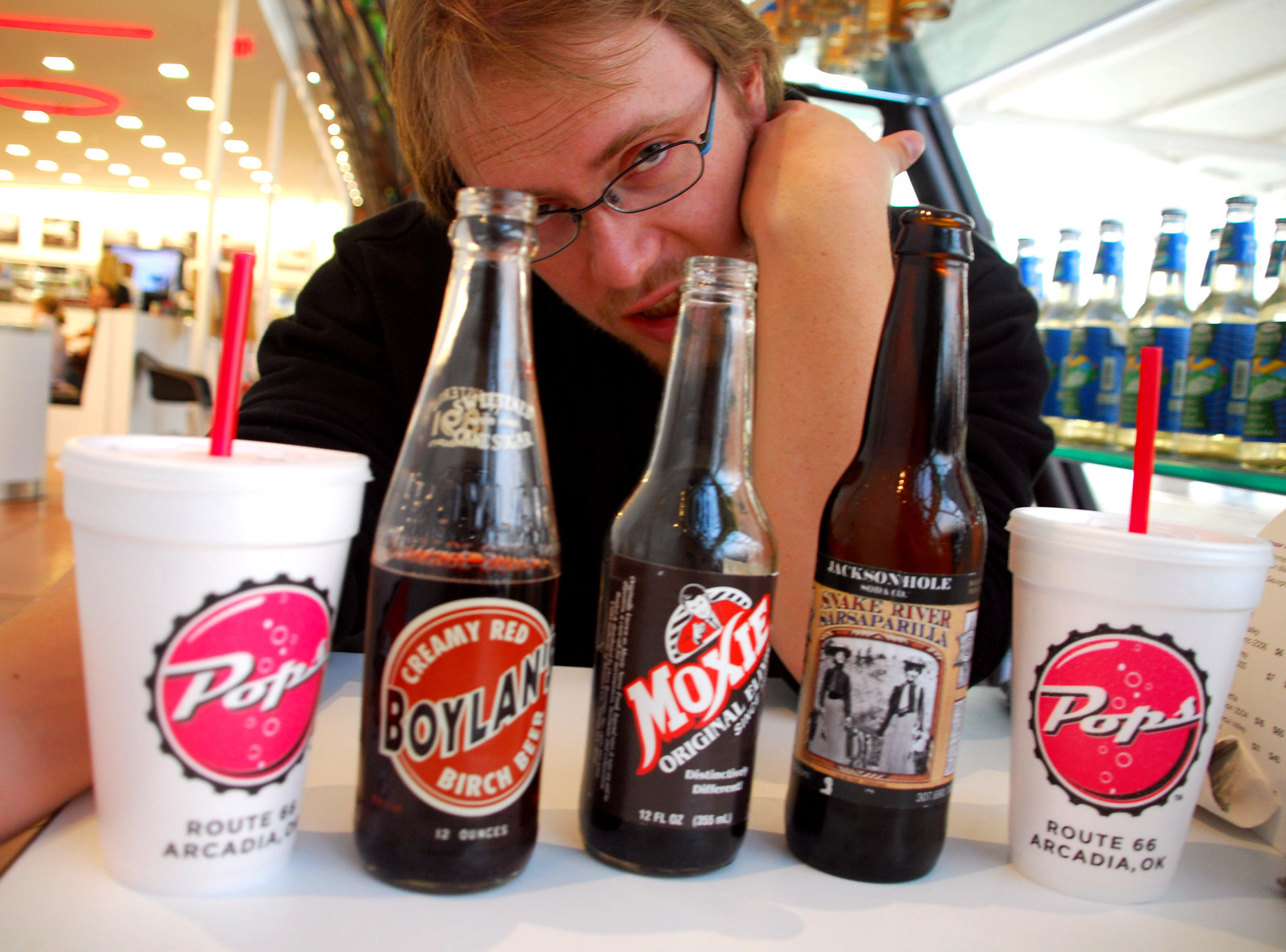A young man with fair skin, dirty blonde hair, and eyeglasses sits at a white table inside a tourist attraction, possibly a restaurant or café. He is casually leaning on the table with his elbow, wearing a short-sleeved black shirt. In front of him, arranged meticulously on the table, are three soda bottles and two identical styrofoam drink cups each adorned with a red bottle cap graphic that reads "POPS" in white letters. Below the bottle cap, in black letters, are the words "Route 66, Arcadia, Oklahoma." Each cup has a red straw protruding from the top. The soda bottles, positioned between the cups, feature various labels: the one on the left says "Boylan Creamy Red Birch Beer" and is about half full, the middle bottle is labeled "Moxie," and the bottle on the right reads "Jackson Hole Snake River Sarsaparilla." Behind him, a display of coolers filled with more soda bottles and a checkout counter can be seen. The setting, filled with the colors red, white, and various shades of glass, evokes a nostalgic atmosphere reminiscent of classic American road trip culture.